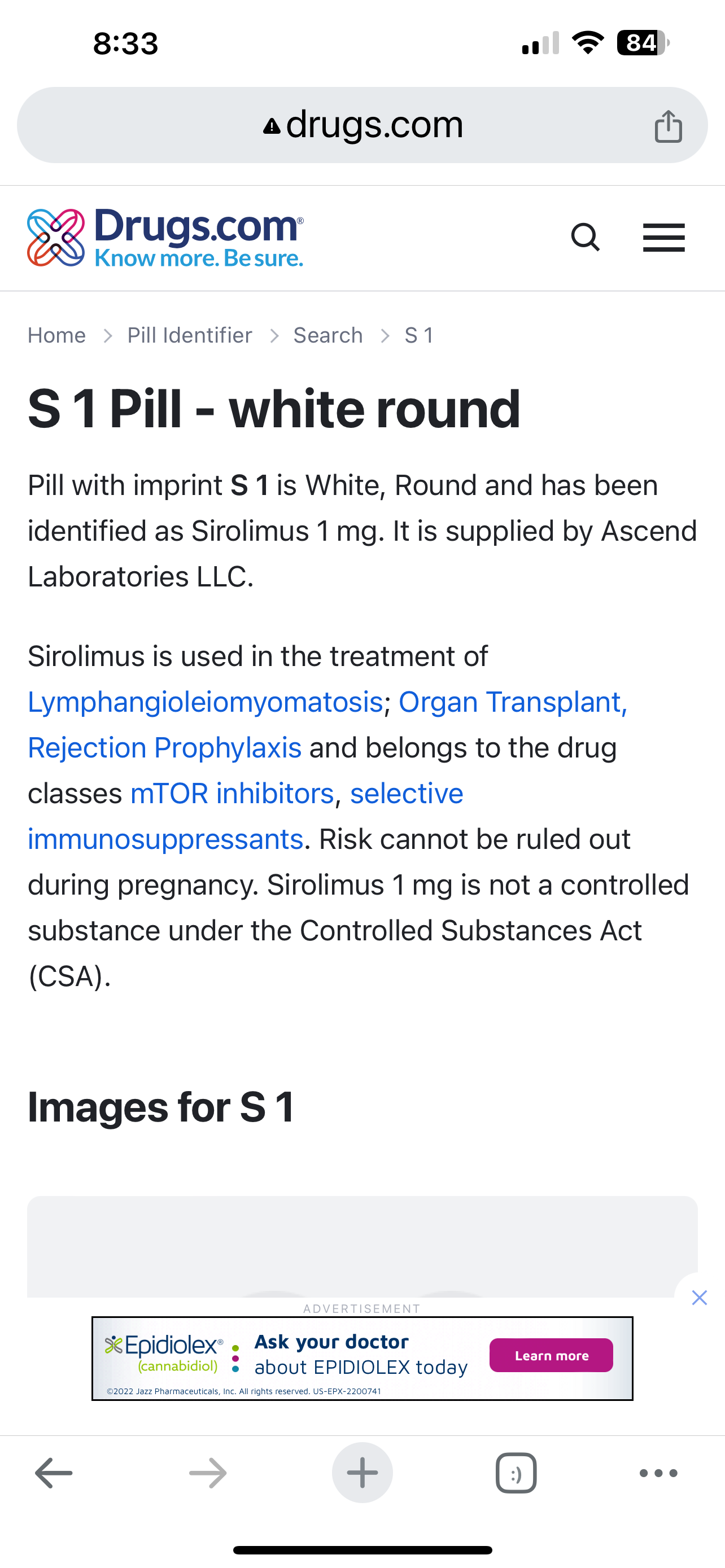Detailed Caption for Screenshot from Drugs.com:

The screenshot depicts the Drugs.com website viewed on a smartphone. In the top left corner, the time reads 8:33, while the top right corner displays the icons indicating strong cellular signal, full Wi-Fi connectivity, and an 84% battery charge.

Directly below the status bar, there is a search field with the text "drugs.com" entered. To the left of the search field, the Drugs.com logo is displayed, followed by the tagline "No more, be sure." On the right side of the search bar, there is a search icon and a menu icon consisting of three stacked horizontal lines.

Beneath the search field, a navigation bar features categories labeled "Home," "Pill Identifier," "Search," and "S1." Below this bar, the main content of the screen begins with a title in large font: "S1 Pill, White, Brown."

The description details the pill imprinted with "S1," specifying that it is white and brown in color. The pill has been identified as Sirolimus, 1 mg, supplied by Ascend Laboratories, LLC. The information highlights Sirolimus' uses, which include treatment of lymphangioleiomyomatosis and prophylaxis for organ transplant rejection. It belongs to the drug classes of mTOR inhibitors and selective immunosuppressants. All medical terminologies and drug classifications appear in blue text.

A note indicates that Sirolimus is not classified as a controlled substance under the Controlled Substances Act (CSA). Below this description, there is a section labeled "Images for S1," followed by a gray bar that demarcates the end of this segment and the start of another section.

The overall layout and presentation make it easy to navigate and understand the detailed drug information provided.